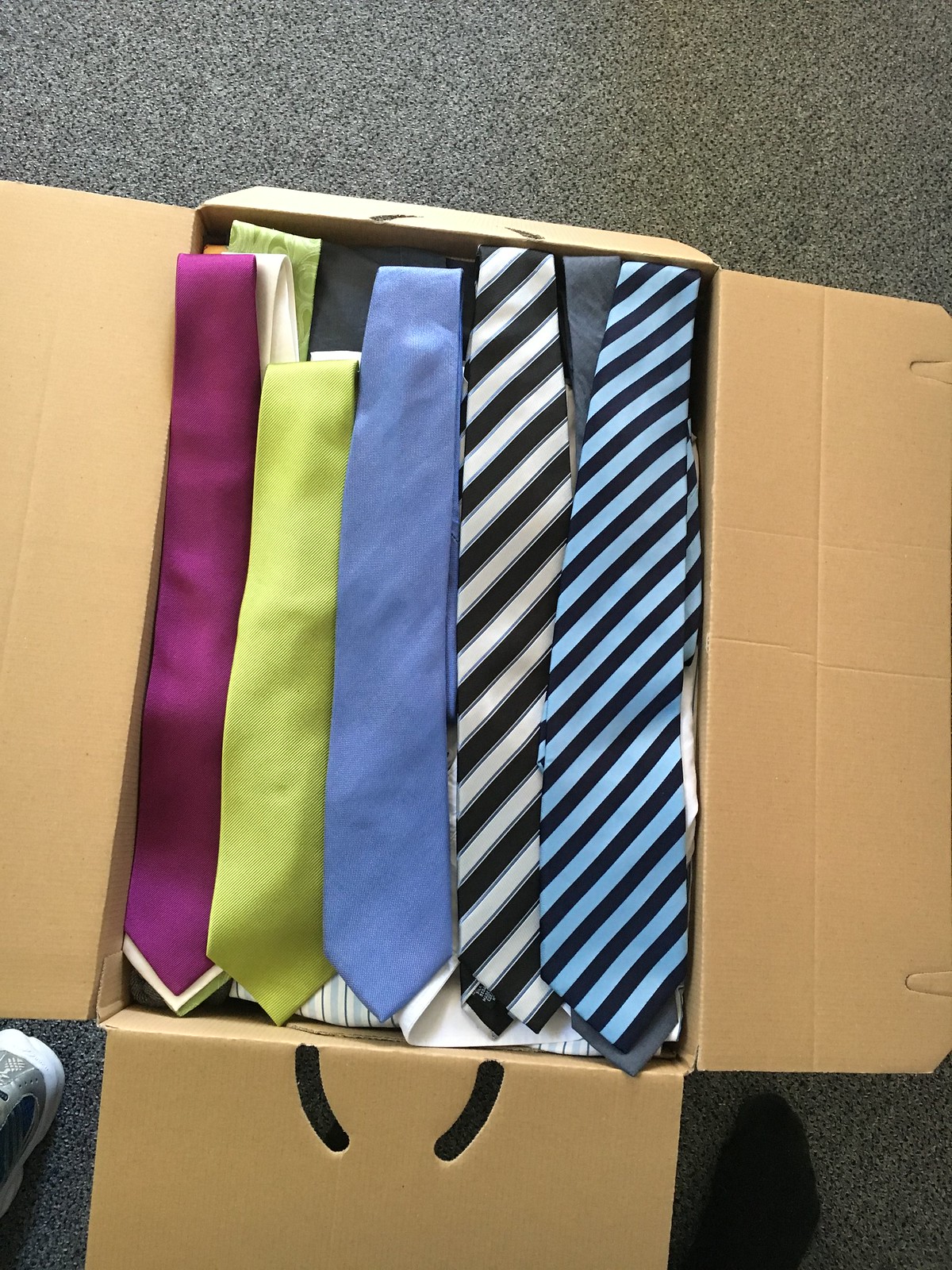This image captures a detailed top-down view of a light brown, open cardboard box filled with neatly folded neckties, positioned on a gray carpet. You can glimpse the tips of gray and white sneakers and a foot clad in a black sock at the edges of the frame. Arranged in a horizontal row on the top of the pile are five distinct ties: a maroon tie on the left, followed by a lime green tie, a solid light blue tie, a black and white striped tie, and finally, a tie featuring light blue and black diagonal stripes. Beneath these visible ties, more ties are layered, and there appears to be a hint of a striped shirt. The varied descriptions emphasize the visual clutter and abundance of ties, creating a vivid portrayal of the contents within the box.